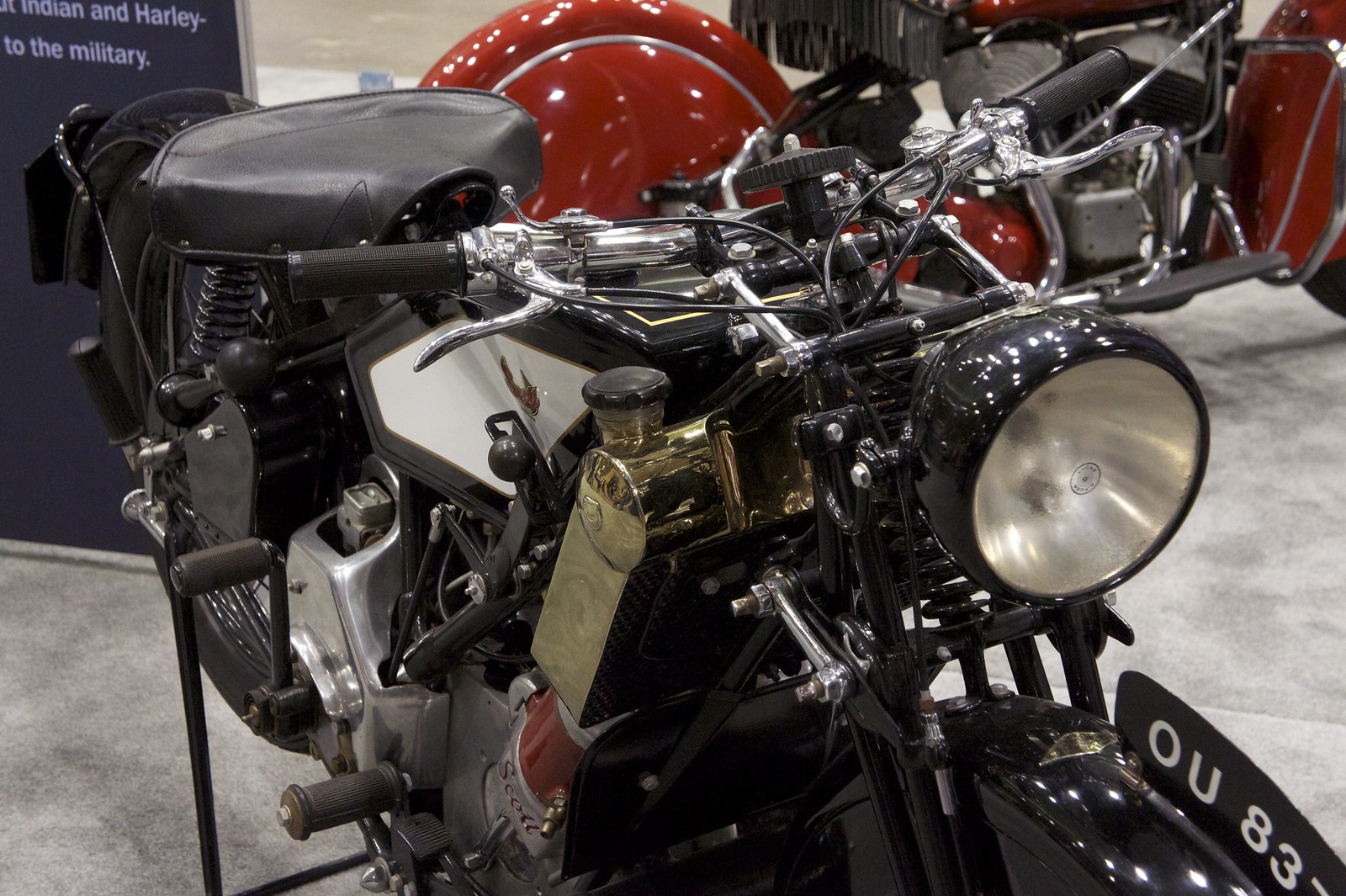This detailed image captures the front view of a vintage motorcycle, likely part of a museum exhibit. The motorcycle is predominantly black, featuring a large, round headlight with a clear silver interior and a black lens. The fenders, both front and rear, are black, as is the one visible tire. The black seat appears to be made of leather, complemented by black spring supports.

Engraved on the silver engine, the name "S. Scott" stands out, though its significance—whether it be the owner's name, the make of the motorcycle, or a component brand—remains uncertain. The fuel tank is a striking cream color with white and black trim, and the handlebars are chrome with black grips.

In the background, a red ball and various signs are visible, including a partially cut-off dark navy blue sign that reads, "Harley to the military." The setting appears to be indoors, likely a showroom or garage, characterized by a white floor and walls painted blue. Additional equipment and billboards suggest the space is used for display purposes. A notable detail is a black license plate on the front fender, displaying the text "OU83" in white lettering.